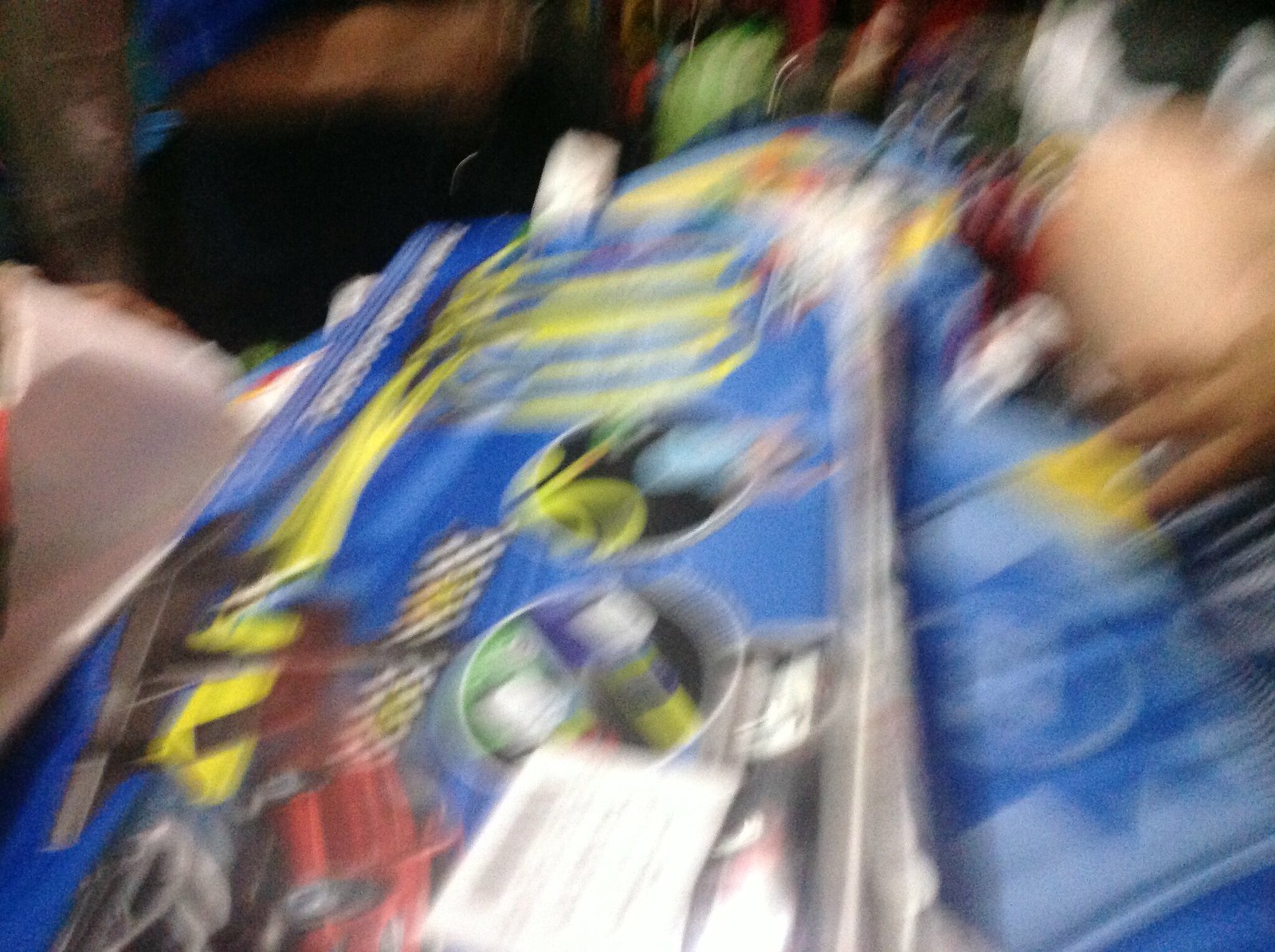This extremely blurry color photograph captures a scene that is difficult to discern with clarity. In the upper right corner, there are vague, human-like shapes and what appears to be part of a hand. Dominating the center is a large blue and yellow object, likely a table adorned with a tablecloth. The tablecloth features an icon resembling a race car. On the table, one can make out several silver dishes containing unidentifiable items. The upper left corner of the image is dark and features black and brown hues. There is no legible text, and no fully visible people, animals, plants, flowers, trees, or buildings present in this photograph.